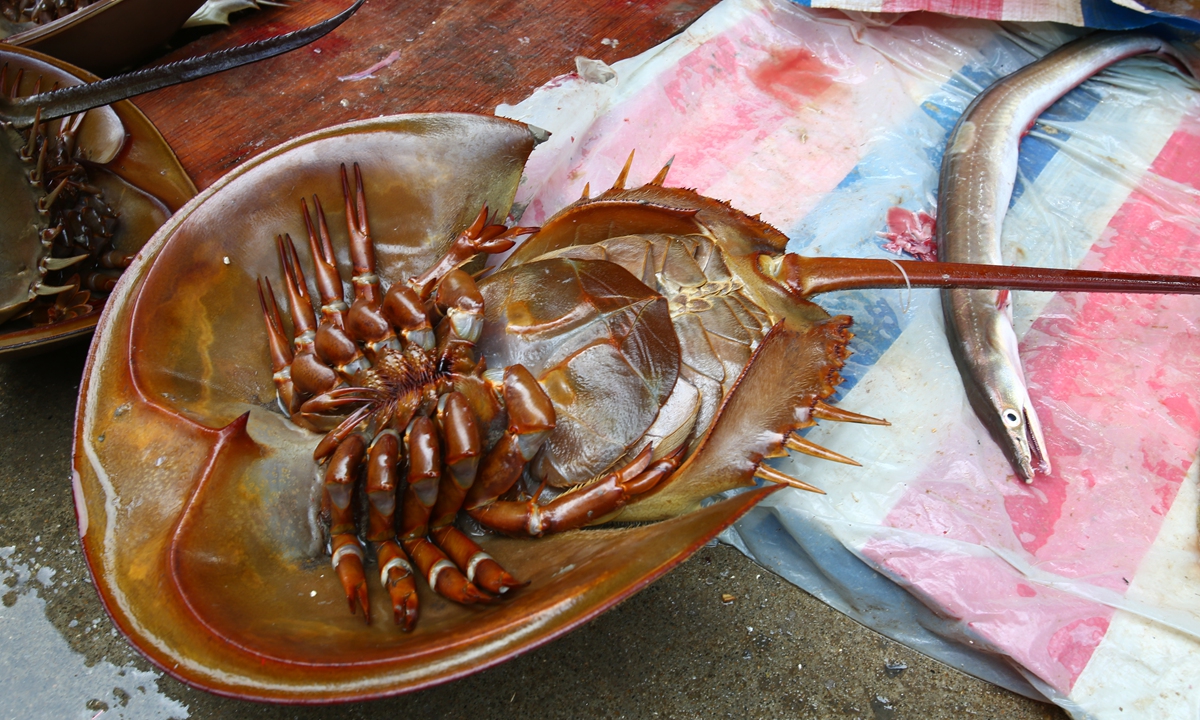This detailed photograph (or possibly a drawing) captures a captivating scene of sea creatures displayed on a wooden table. Dominating the center is a large, upside-down horseshoe crab, showcasing its brownish, shiny shell and eight legs splayed outwards. Its long, pointed tail stretches behind it. Another horseshoe crab, also turned upside-down, is placed to the left of the main one. To the right of the large horseshoe crab lies an eel-like fish, distinguishable by its slender form and open mouth, resting on a red, blue, and white striped cloth. The setting appears to be near the shore, with some sand visible at the bottom of the image. The overall tones are earthy, with hues of brown and gray, suggesting either a faded photograph or a meticulously detailed painting.